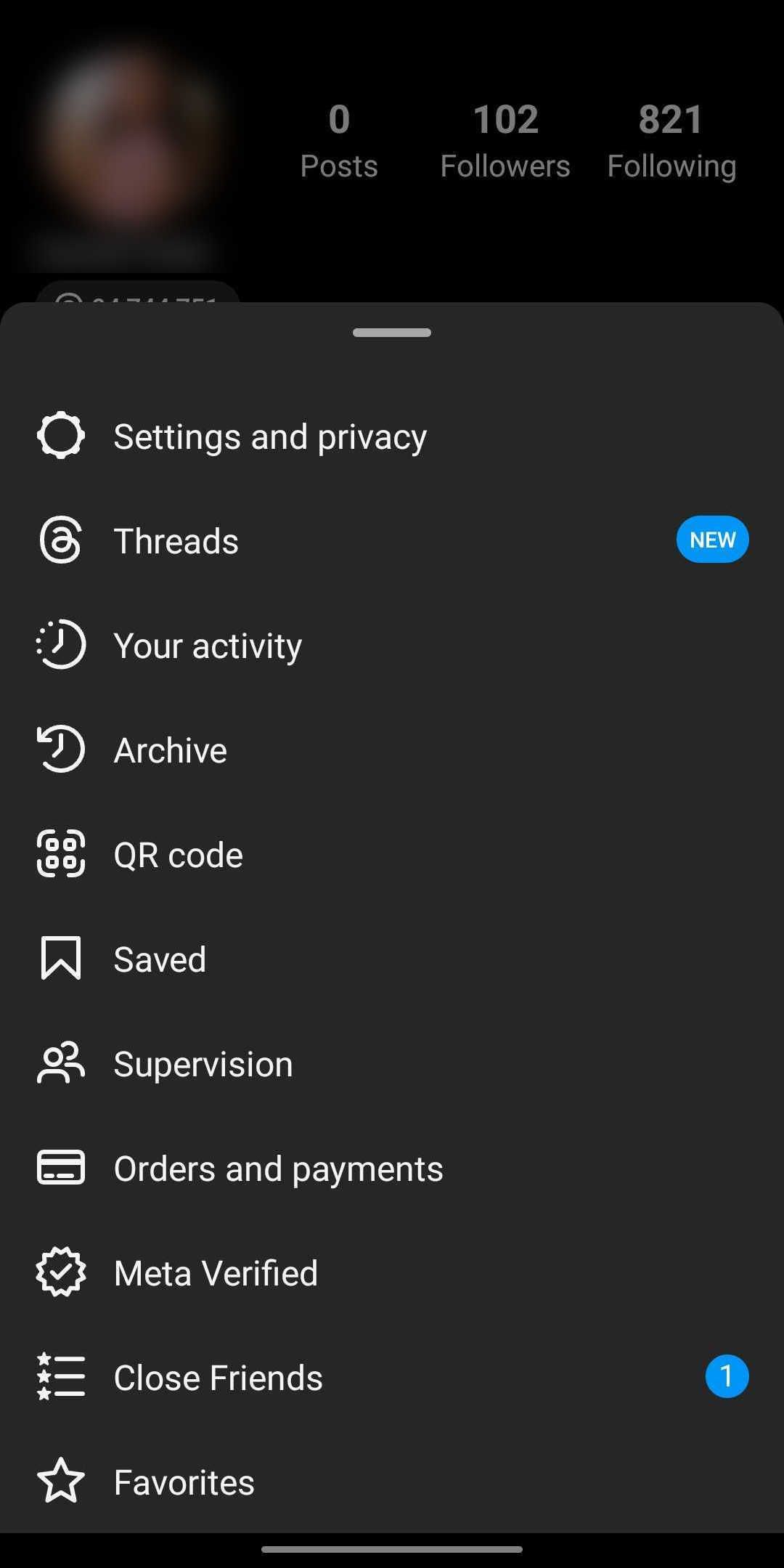The image shows a smartphone screen with a dark theme interface, primarily in black tones. At the very top of the screen, there's a blurred profile picture, next to which the text indicates "0 posts," "102 followers," and "821 following," suggesting it could be a social media platform like Twitter or X.

Below the profile section, occupying about three-quarters of the image, is a menu. This menu appears similar to what you would see when sliding up a settings or options panel on a smartphone. The menu contains the following items listed with their respective icons:

1. **Settings and Privacy** - Represented by a gear icon.
2. **Threads** - Represented by a thread icon with a "new" label next to it.
3. **Your Activity** - Indicated by a clock icon.
4. **Archive** - Indicated by a clock and arrow icon.
5. **QR Code** - Accompanied by a QR code icon.
6. **Saved** - Represented by a bookmark icon.
7. **Supervision** - Depicted with an icon of two people.
8. **Orders and Payments** - Shown with a Visa card icon.
9. **Meta Verified** - Indicated by a checkmark icon.
10. **Close Friends** - Represented by a list with stars icon and has a blue bubble with a "1" on the right side.
11. **Favourites** - Shown at the bottom with a star icon.

The blue bubbles on the screen highlight notifications or new elements: one next to "Close Friends" marked with "1" and another next to "Threads" labeled as "new."